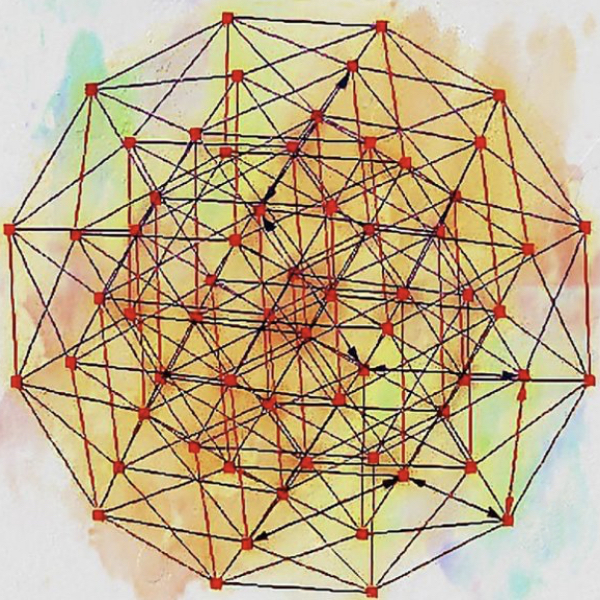The photograph depicts a complex geometric design resembling a busy, interconnected network of red dots and lines, forming a 12-sided, spherical, or ball-like shape that is reminiscent of a geodesic structure. The lines—primarily red with interspersed black—radiate and connect in various directions, creating an intricate web of geometrical patterns that includes a noticeable cross-hatching effect. The design sits against a watercolor-painted background featuring smudges of light green, yellow, orange, light blue, pink, white, and purple, giving the backdrop a soft and irregular appearance. The image measures five by five inches and maintains a purely abstract nature with no visible title or artist attribution. Black arrows are scattered within the composition, pointing in various directions, adding to the dynamic visual complexity of the piece.